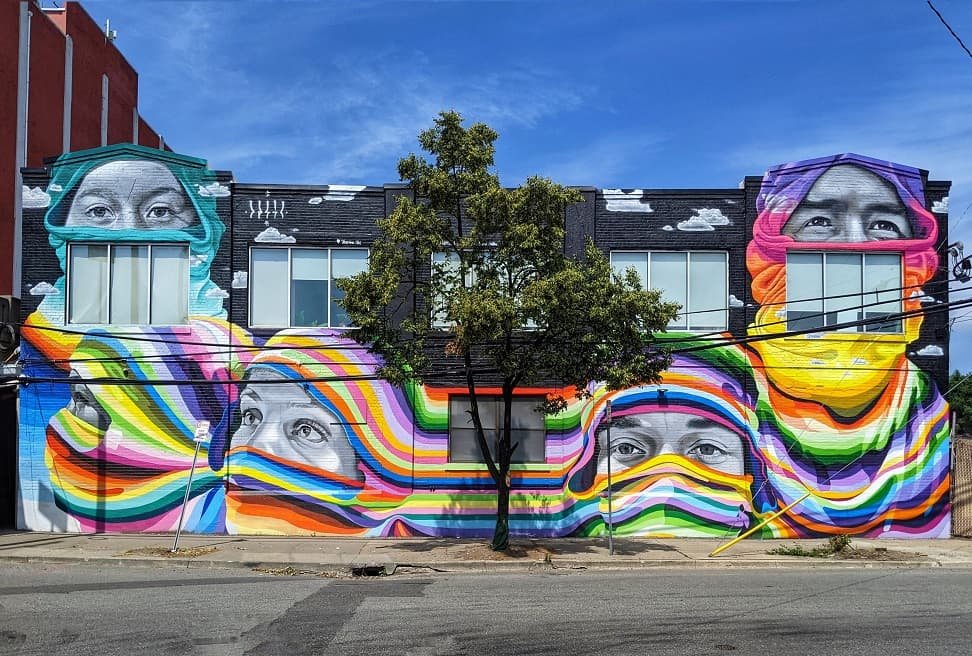The image depicts a two-story, dark grey brick building with a wall fully adorned in graffiti art. The artwork spans five sections of the wall, showcasing five distinct grey faces, each adorned with vibrant, multicolored facial and head coverings in striped patterns of blue, yellow, and orange. The faces are positioned with two on the left, one in the center, and two on the right. A tree with dark green leaves grows from the sidewalk, standing prominently in the middle of the mural. The building features three-pane windows on the upper floor, with three of them shut, and a smaller, divided window on the ground floor. The scene is set against a backdrop of a clear blue sky with minimal clouds, a sidewalk, and a quiet street with no pedestrians present.